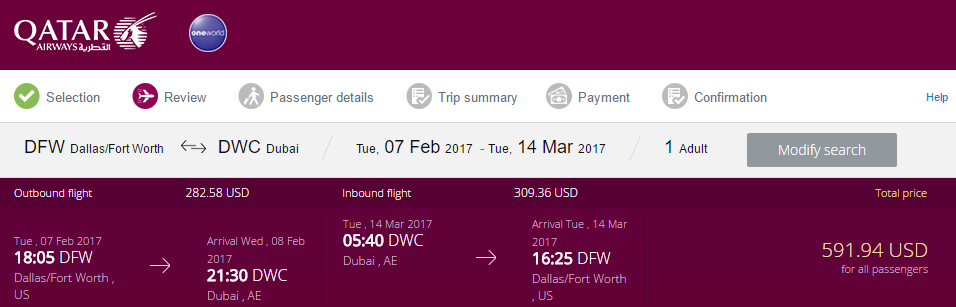**Detailed Caption:**

This screenshot from the Cape Cutter Airways booking system features a prominent maroon box at the top labeled "Cape Cutter Airways." Below this, a blue circle indicates that the selection is "One Way." The interface includes a selection process checklist with items such as "selection" (marked with a green check), "review" (signified by a maroon circle featuring a plane icon), "passenger details," "trip summary," "payment confirmation," and "help."

The journey details indicate a flight from Dallas-Fort Worth to Dubai on Tuesday, February 7, 2017, returning on March 14, 2017. The booking is for one adult traveler. 

The outbound flight departs from Dallas-Fort Worth on Tuesday at 6:05 PM, arriving in Dubai on Wednesday at 9:30 AM, with a ticket price of $282.58. The return flight leaves Dubai on Tuesday, March 14th at 5:40 AM and arrives back in Dallas-Fort Worth at 4:25 PM the same day, costing $309.36. The total cost for the round trip amounts to $591.94 USD.